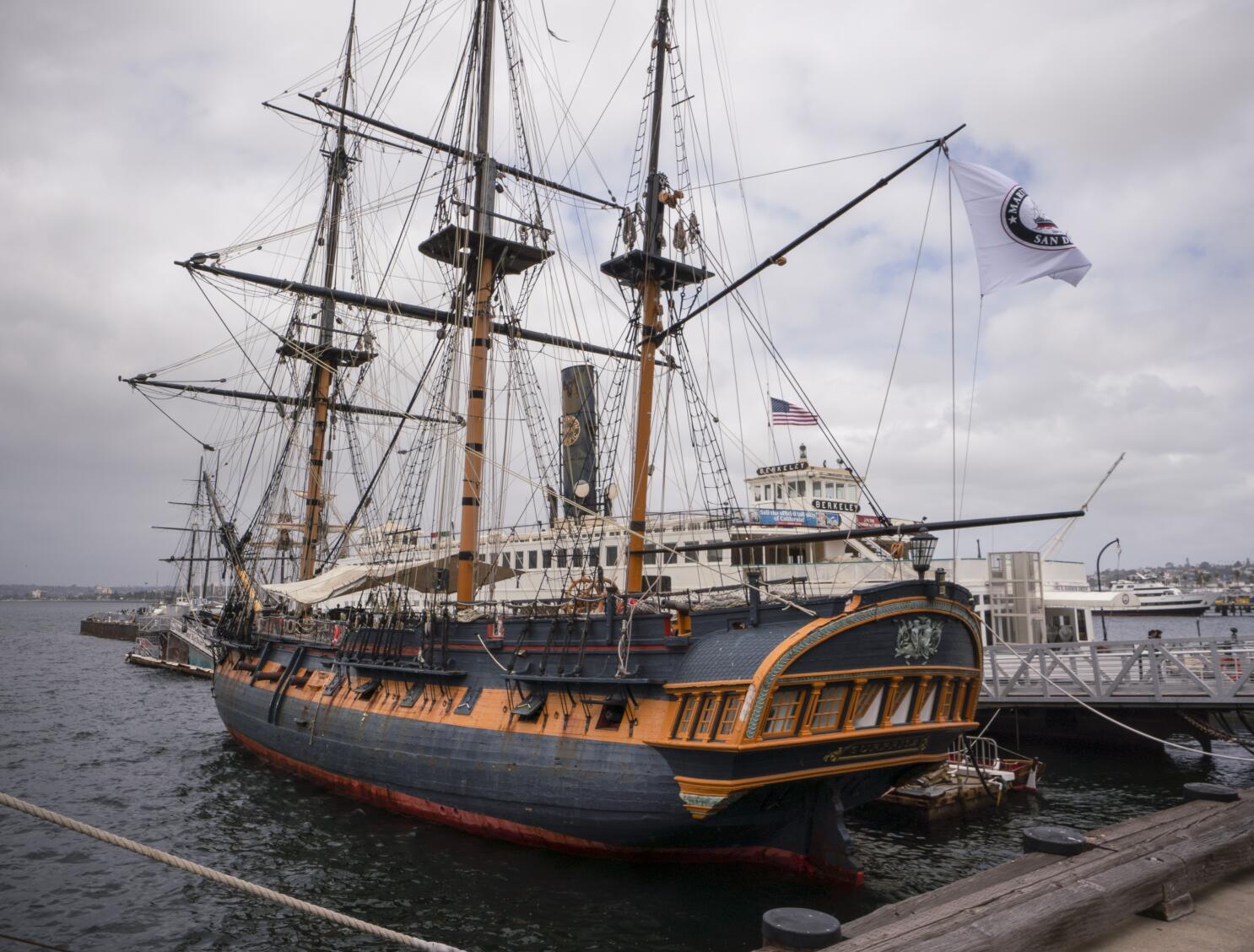This image depicts a large, old-fashioned wooden sail ship docked alongside a concrete sidewalk. The vessel features a distinct red layer at the bottom, transitioning into black and brown hues, with another black section above. Although the ship's sails are not hoisted, numerous masts rise skyward, each equipped with platforms where a person could stand.

On the ship, a large steering wheel is visible, but no people are present. A prominent flag flutters at the rear of the ship, although its details are obscured by the wind. Additional ropes are tethered to the dock, securing the ship in place.

To the right of the primary ship, an assortment of smaller boats can be seen, including one with a large American flag centered on it. The background reveals buildings and other structures, set under a mostly cloudy sky with patches of blue peeking through. The surrounding water appears dark and slightly agitated, suggesting a breezy day. Overall, the scene conveys the historical charm and robust construction of the old-timey sail ship, hinting at its potential use for cruises or similar activities.